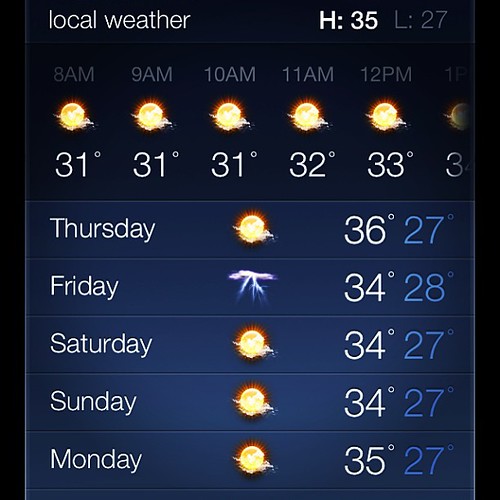This digital image depicts the local weather forecast. On the right side, temperature details are provided: a high of 35 and a low of 27 degrees. Hourly temperature readings are listed as follows: 8 AM - 31 degrees, 9 AM - 31 degrees, 10 AM - 31 degrees, 11 AM - 32 degrees, and 12 PM - 33 degrees.

The extended forecast includes:
- **Thursday**: A bright sun symbol indicating clear weather with a high of 36 degrees and a low of 27 degrees.
- **Friday**: A thunderstorm symbol suggesting stormy weather with a high of 34 degrees and a low of 28 degrees.
- **Saturday**: A sun symbol again indicating clear weather with a high of 34 degrees and a low of 27 degrees.
- **Sunday**: Another sun symbol representing clear conditions with a high of 34 degrees and a low of 27 degrees.
- **Monday**: Yet another sun symbol for clear weather with a high of 35 degrees and a low of 27 degrees.

The information is clearly laid out to provide a comprehensive view of the upcoming weather conditions.